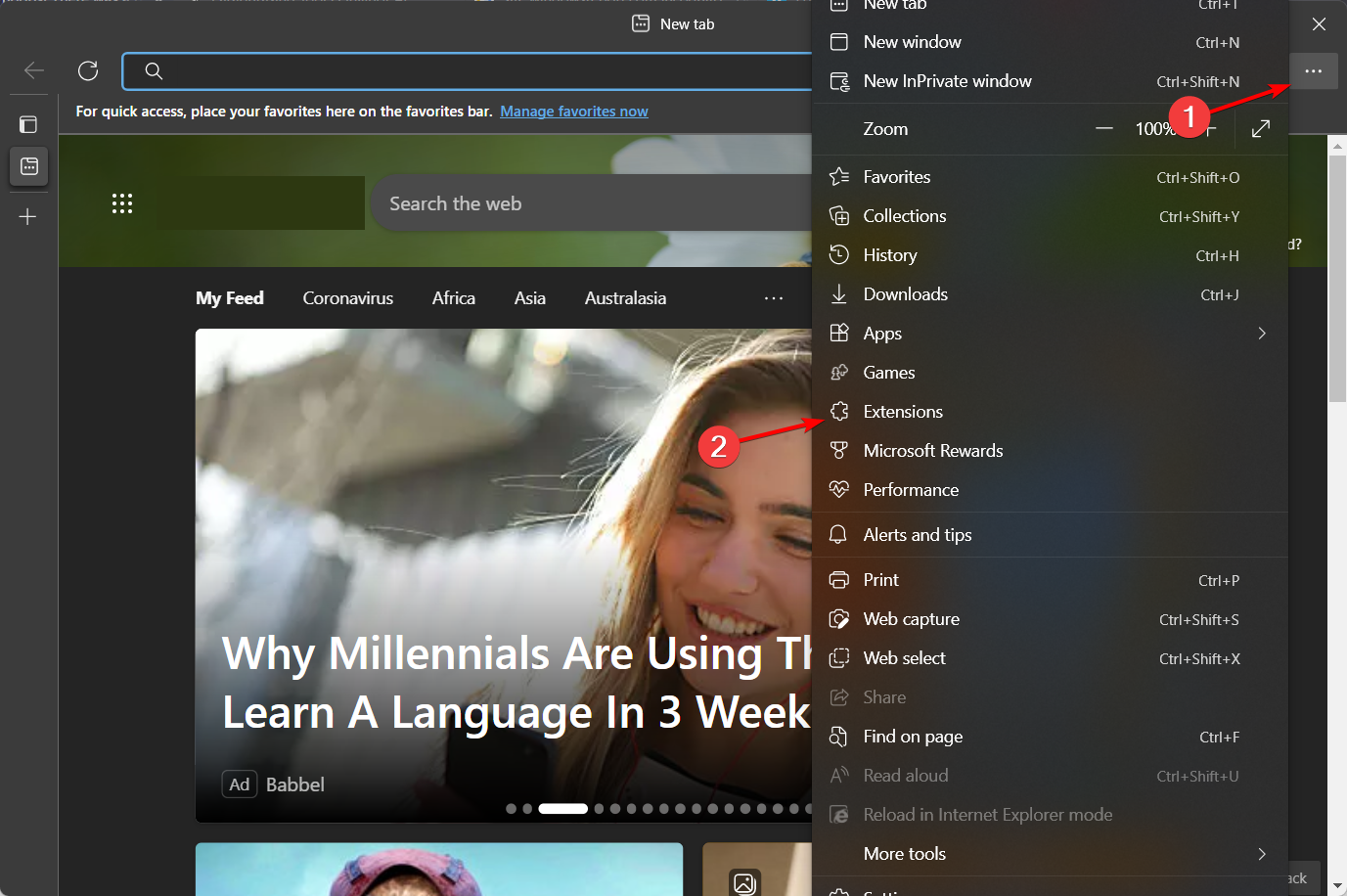This image is a detailed screenshot intended for a how-to guide. Captured from a Windows computer, it displays the Microsoft Edge browser, specifically its Bing homepage. The predominant colors in the background are shades of gray and dark gray. At the top of the browser window, the label "New Tab" is visible. Central to the image are two or three color images representing articles in the "My Feed" section, confirming that this is the Bing start page.

A dropdown menu is open on the screen, featuring two highlighted items marked with red circles and numbered arrows. The first highlighted area, labeled with the number "1", points to the three-dot menu icon located at the upper right-hand side of the browser. The second highlighted area, labeled with the number "2", points to the "Extensions" option within the dropdown menu. This visual guide implies instructions for changing, adding, or removing extensions in the Microsoft Edge browser. Additionally, there are several small, indeterminate icons situated on the far left of the window, further suggesting a comprehensive view of the browser's interface. Overall, this is an instructional screenshot showing how to manage browser extensions in Microsoft Edge.